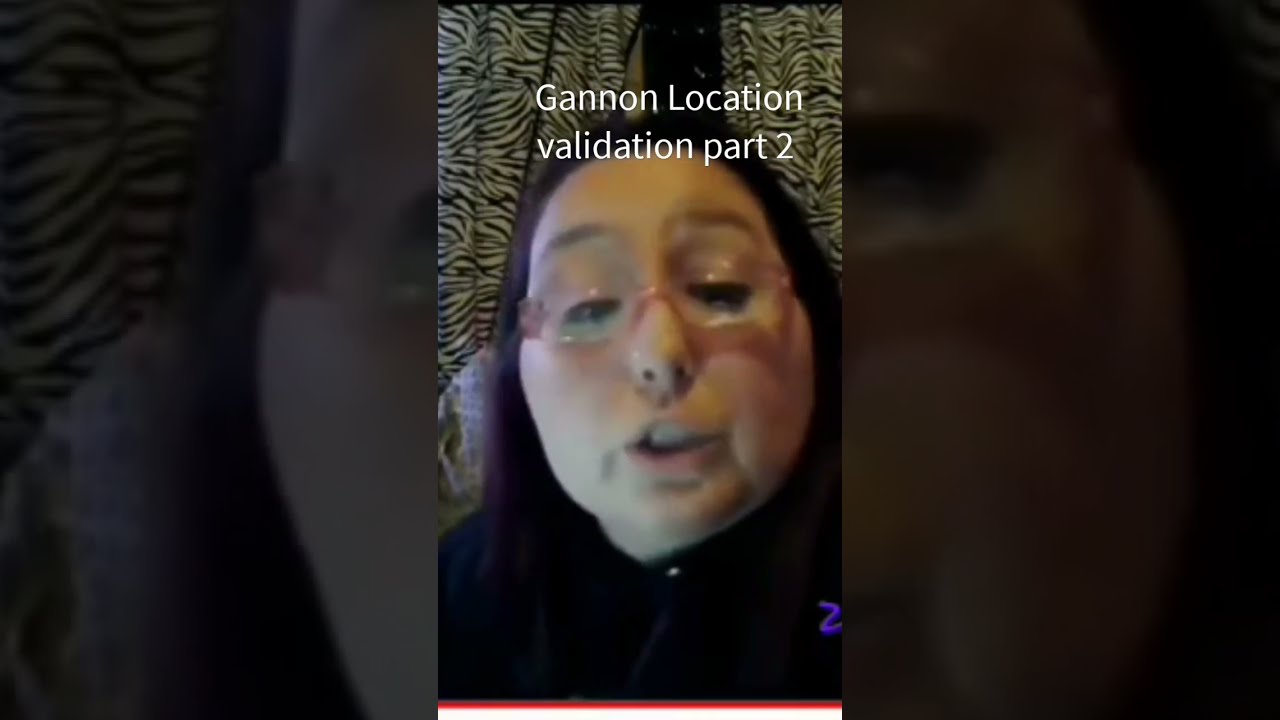The image is a composite split into three sections: the left, center, and right. The central portion features an indoor selfie of a young, light-skinned, heavier-set female with a rounded face and straight, dark brown hair. She wears light pink plastic-framed glasses and a dark black high-necked shirt adorned with a small "Z" logo. Her expression captures her in mid-sentence, with her eyebrows raised and her mouth open. Above her head, the text "Gannon Location Validation Part 2" is visible in white print. The left and right sections of the image are magnified and darkened portions of her face, highlighting the left and right sides respectively. The backdrop consists of zebra-patterned curtains, providing a distinct setting. The image, slightly blurry, includes only the woman's face and part of her upper body.